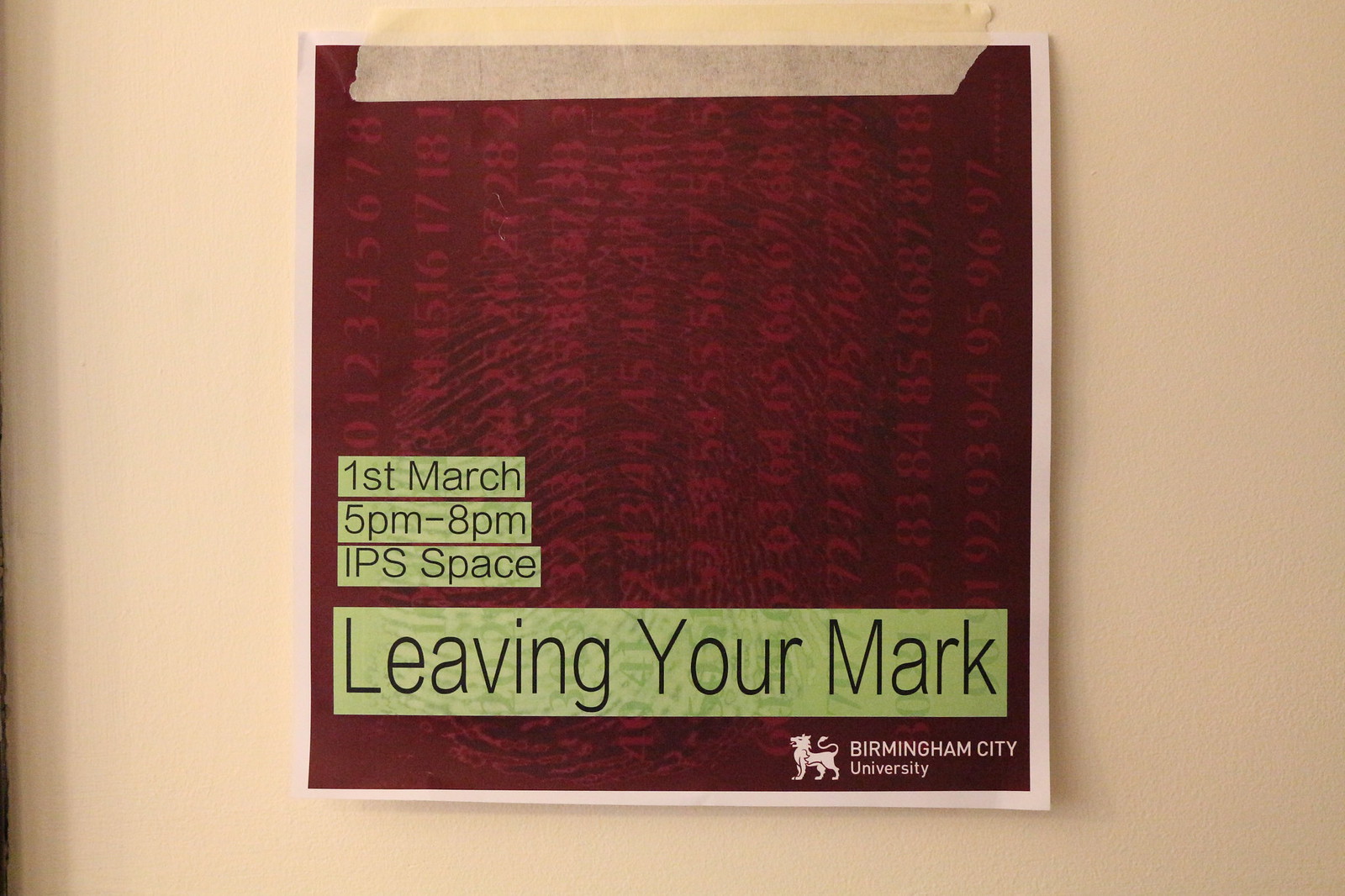This is a photograph of a poster attached to a beige wall using a large, translucent piece of tape running horizontally across the top, blending with the beige wall. The poster itself is brown with a faded, textured pattern of numbers in the background. It features a beige border that matches the wall. Prominently displayed on a green rectangular background within the poster are the details: "1st March," "5 p.m. to 8 p.m.," and "IPS space." Below these details, in the largest font, is the event title "Leaving Your Mark." In the lower right corner, the poster bears the logo and text of "Birmingham City University," accompanied by a small sigma symbol of a lion. The colors in the poster include shades of tan, maroon, red, green, black, and white, with the overall design centered within the image, capturing the essence of a university setting.